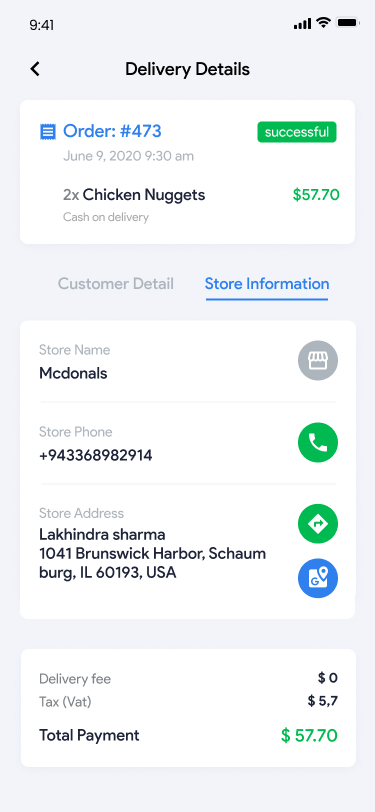Here's a cleaned-up and detailed caption for the given image:

---

The screenshot displays detailed information regarding a food delivery order from McDonald's. At the top left corner, the time is shown as 9:41 AM. Centered below is the heading "Delivery Details." Further down, in blue text, is "Order number 473" with the date and time specified as "June 9th, 2020, 9:30 AM." A green button on the right of the screen indicates that the order was "Successful."

The items ordered consist of "2x chicken nuggets." The payment method is indicated as "Cash on Delivery," with the total cost displayed in green, "$57.70." On the right side of the screen, a blue tab labeled "Store Information" can be seen.

Under "Store Information" on the left, the following details are listed:
- "Store Name: McDonald's"
- "Store Phone: 94-336-8982-914"
- "Store Address: Lechendra Sharma, 1041 Brunswick Harbour, Schaumburg, IL 6193, USA"

Additional cost information includes:
- "Delivery Fee: $0.00"
- "Tax: $5.70"
- "Total Payment: $57.70"

---

This caption describes all available data points from the screenshot, reconstructing them into a coherent and detailed summary.